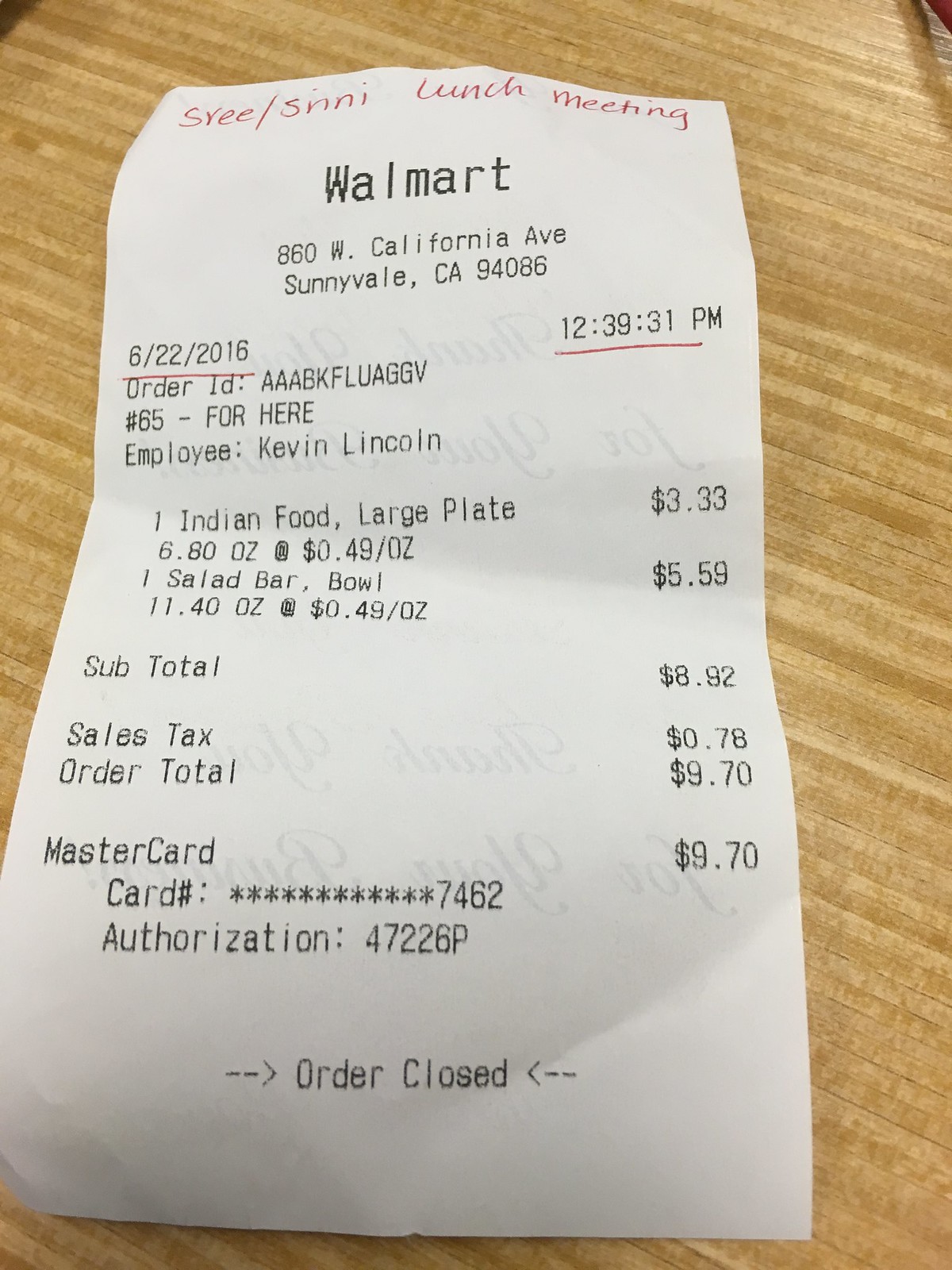The image depicts a white Walmart receipt laid on the center of a wooden table characterized by alternating vertical light brown and medium brown thin stripes of wood. At the top of the receipt, written in red ink, is "SYEE/SINNI lunch meeting," with portions of the receipt underlined in red. The receipt is from the Walmart located at 860 West California Avenue, Sunnyvale, California, 94086. The printed details include the date 6-22-2016 and time 12:39:31 PM. The order, identified with the ID AAABKFLUAGGV and marked "for here," was processed by employee Kevin Lincoln. The items listed are one large plate of Indian food priced at $3.33 and a salad bar bowl priced at $5.59, totaling $9.70, which was paid for with a MasterCard. The total amount includes a subtotal of $8.92 and a sales tax of $0.78. The MasterCard transaction is noted with card number ending in 7462 and authorization number 47226P. At the bottom of the receipt, it states "order closed."